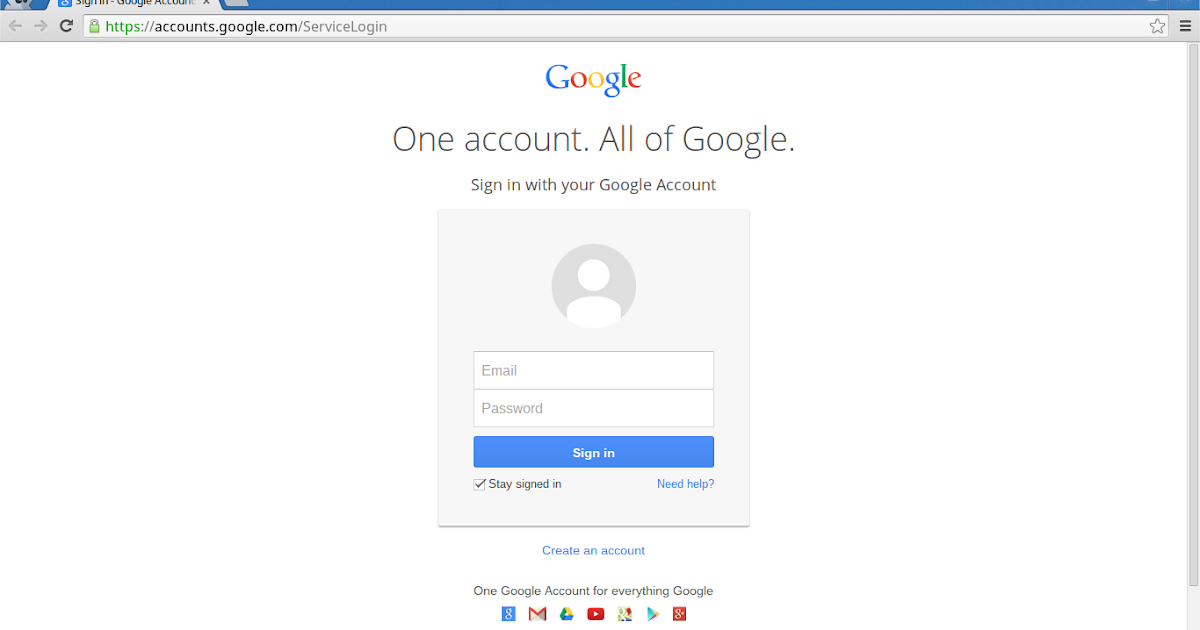This image is a cropped screenshot of a browser page, specifically the sign-in page for Google accounts. The left, bottom, and top edges of the image are cropped, with the visible portion featuring the bottom part of one open tab on the top left. Below the tab is the browser's URL bar stretching across most of the top section, indicating that the webpage is accounts.google.com.

The page itself has a white background. At the top center, the Google logo is prominently displayed. Beneath it, in uppercase letters, is the statement "ONE ACCOUNT. ALL OF GOOGLE." followed by the phrase "Sign in with your Google Account" in smaller text. The main content is a large thumbnail representing the Google login interface. This is depicted as a gray square containing a circular profile picture placeholder. Below the placeholder are two text boxes: one for the email address and one for the password. 

At the bottom of this login interface is a large blue "Sign In" button. To the left of this button, in small black letters, it says "Stay signed in" next to a checked checkbox. To the right of the button, in blue hyperlinked text, it says "Need help?". Below the login interface, there's a prompt in small blue letters saying "Create an account."